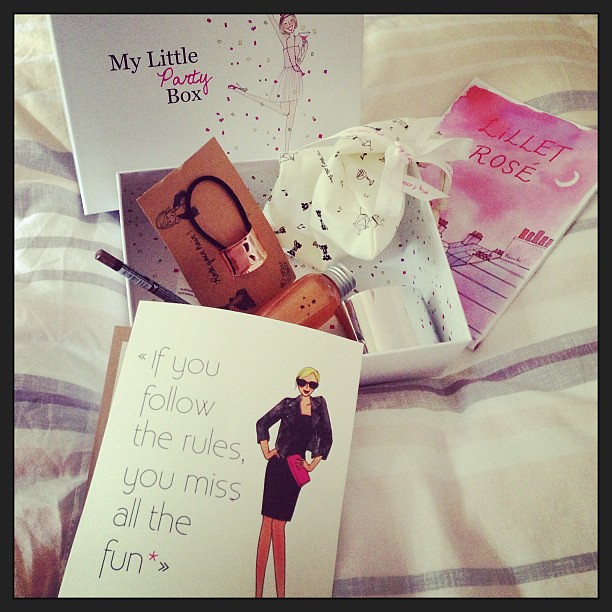The photograph captures a top-down view of a bed with a light beige duvet featuring gray and purple horizontal stripes. Centered on the bed is an open white cardboard box labeled "My Little Party Box" on the lid, which lies above and to the left of the box. The lid showcases a cartoon of a woman in a dress holding a champagne glass with one leg playfully raised. Inside the box, various women's accessories and makeup items are neatly arranged. Visible items include a bottle with a silver cap, a silver flask, a piece of jewelry (possibly a bracelet or necklace) on a beige card, a white bag adorned with black icons, and a black pencil, likely an eyeliner. 

Surrounding the box are two greeting cards: a white one positioned below the box featuring a cartoon woman in a business suit and glasses, hands on her hips, with the caption "If you follow the rules, you miss all the fun," and a pink card to the right of the box titled "Lilette Rose," accompanied by a pink and purple decorative image. A smaller leaflet, partly visible, is also present within the box, contributing to the overall theme of fashion and beauty.